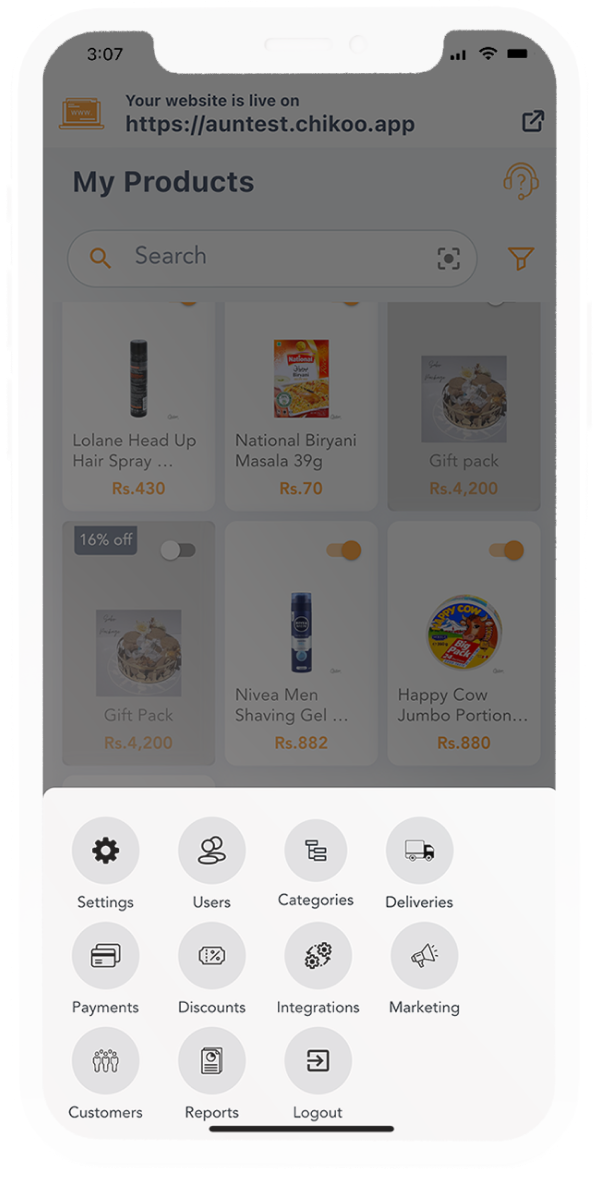The image showcases an app designed for ordering groceries and other food items. The app's website is accessible at antist.chiku.app. At the top of the interface, there's a search bar to help users find specific products. Below the search bar, the layout features a grid of six items, organized in two rows of three. 

The first row includes Lolane Head Up Hairspray, National Biryani Masala Gift Pack—which is marked with a 16% discount—and another unspecified gift pack. In the second row, the items are Nivea Men's Shaving Gel and Happy Cow Jumbo Portion. The shaving gel and Happy Cow products are shown as having been added to the cart, although the cart itself is not visible in the image. Additionally, there are various clickable categories for different product selections available on the app.